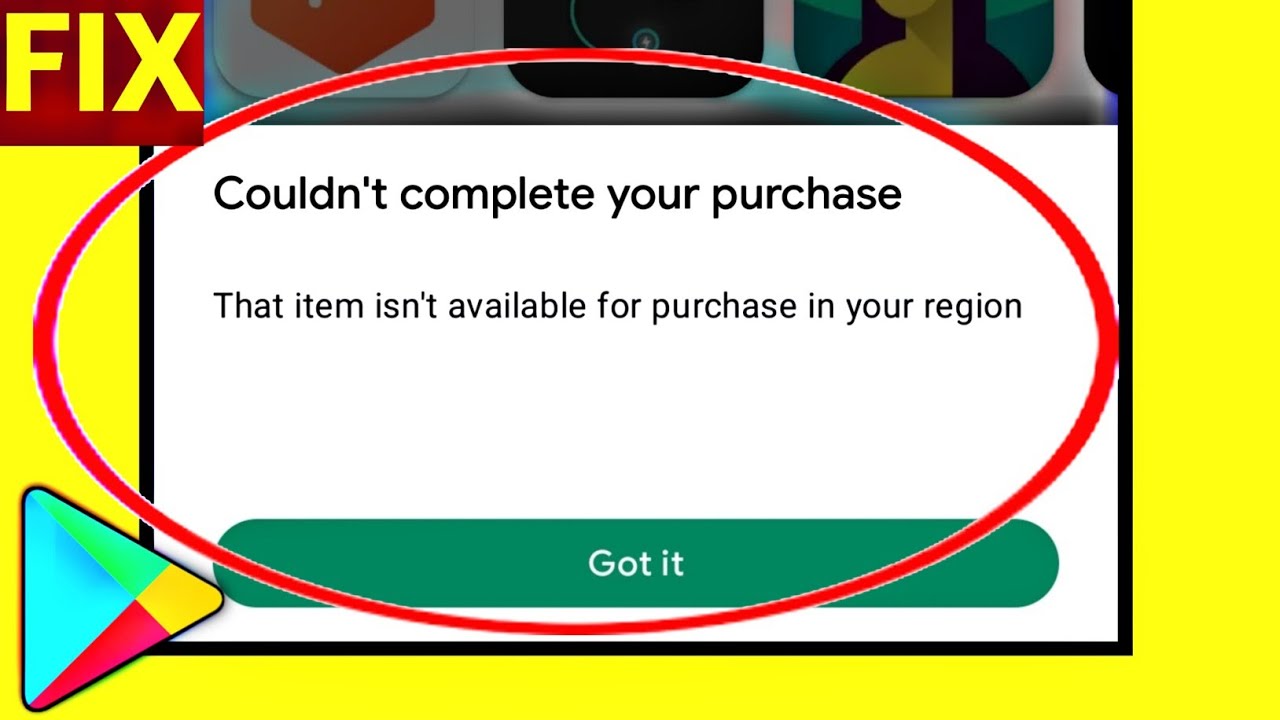The image appears to be a screenshot from an online platform, encapsulated by a yellow border on the sides and bottom. Central to the image is a white rectangle featuring black text that reads, "Couldn't complete your purchase. That item isn't available for purchase in your region." Beneath this message is a large green oval button labeled "Got it." Notably, this entire notification is circled by a prominent red oval.

In the bottom left corner, there is a logo that resembles a Google symbol, composed of a right-facing triangle with sections in blue, green, yellow, and red. 

At the top left corner, the word "FIX" is displayed in yellow letters against a red background.

Additionally, the top section of the image showcases various icon-like buttons reminiscent of those found on a cell phone interface. These include an orange-colored icon and an icon depicting a photo of a person.